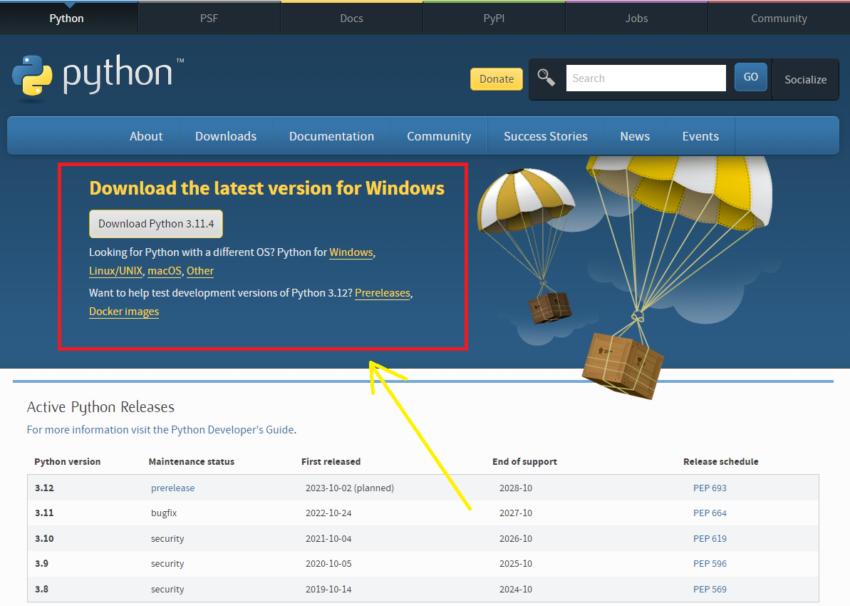The image displays a detailed screenshot of a web page dedicated to Python programming. At the top left, the Python logo and the word "Python" are prominently displayed. Adjacent to the logo, a yellow "Donate" button stands out, followed by a search bar with a "Go" button. The header also contains navigation buttons for various sections including Python, PSF, Docs, Pi, PL, Jobs, and Community.

Below the main header, another set of navigation buttons is arranged, providing quick access to sections such as About, Downloads, Documentation, Community, Success Stories, News, and Events. A notable red box on the left side of the page draws attention with the message "Download the latest version for Windows - Download Python 3.11.4." It also offers options for other operating systems like Windows, Linux, Unix, and Mac OS, and mentions pre-releases and Docker images for Python 3.12.

To the right of this red box, an illustrative graphic features parachutes dropping crates, adding a visually engaging element to the page. At the bottom of the page, there is a chart that details the release dates for various Python versions, providing a quick reference for users interested in the version history.